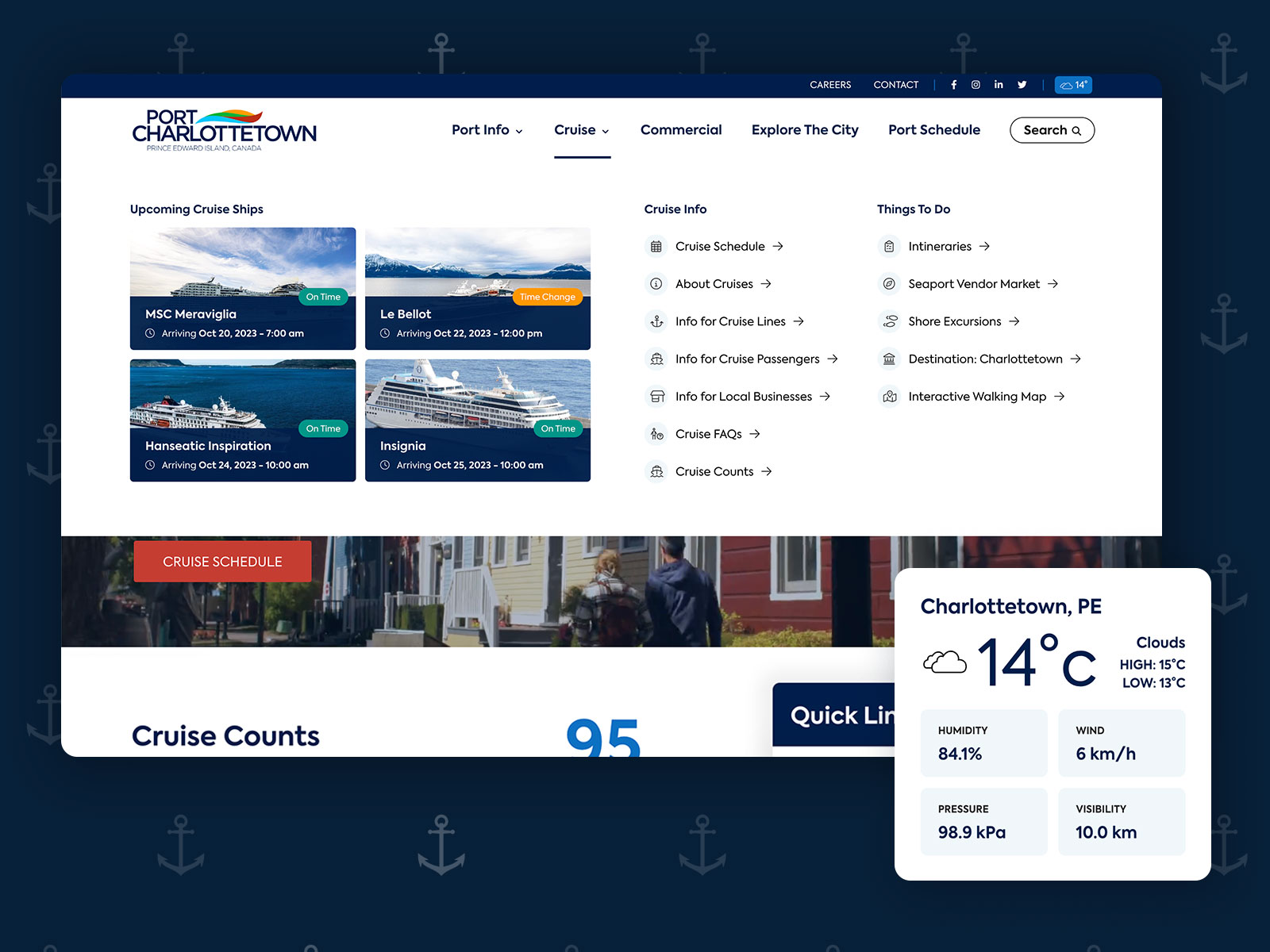**Descriptive Caption:**

This screenshot, presumably taken from an iPad, features a square-oriented display with a navy blue background embossed with a repeating pattern of light gray anchors. Prominently at the top, the webpage header showcases "Port Charlottetown" alongside a navigation bar with clickable dropdown menus labeled: Port Info, Cruise, Commercial, Explore the City, and Port Schedule. The "Cruise" section is selected, as indicated by the underline, revealing images of four distinct cruise ships. Adjacent to these visuals are two informational sections titled "Cruise Info" and "Things to Do," which provide various clickable links for further details. A widget in the lower right-hand corner indicates the current weather in Charlottetown, PE, displaying a temperature of 14 degrees Celsius, with 84% humidity and additional weather data.